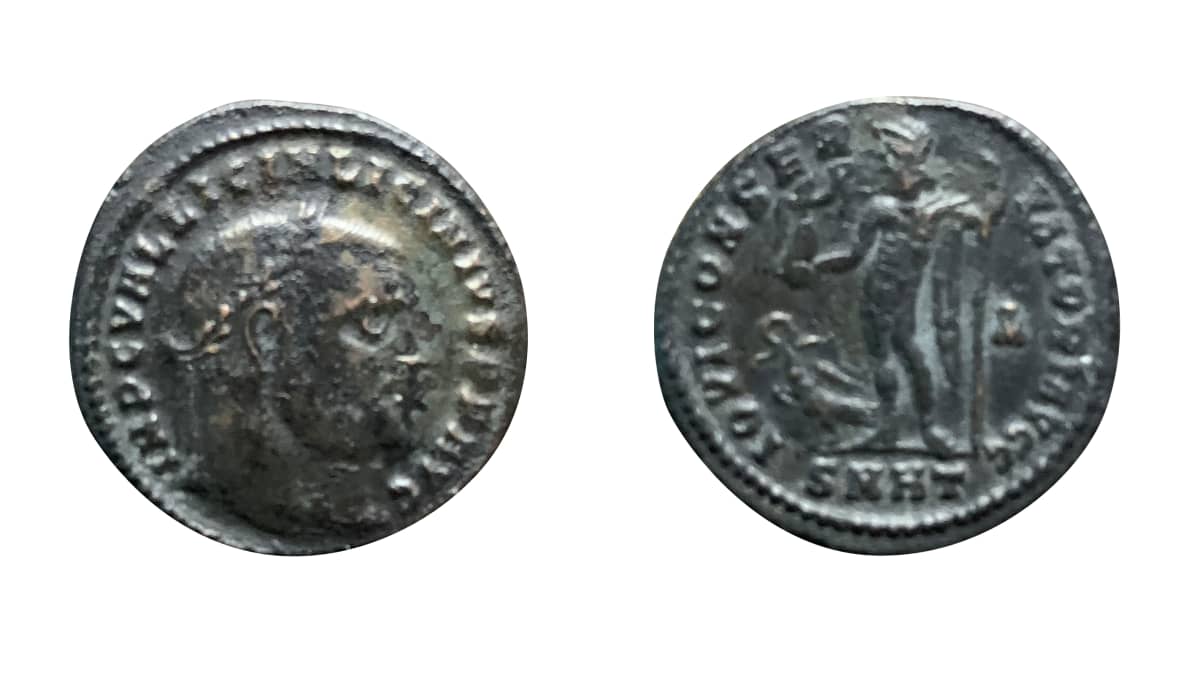The image is a landscape-oriented color photograph featuring an ancient, weathered coin set against a white background. The coin is shown in two side-by-side photographs, with the head side on the left and the tail side on the right. The coin, primarily dark bronze with areas appearing dark gray and greenish from corrosion, has an imperfect circular shape due to its age and wear. 

On the left, the head side depicts a man's right profile adorned with a laurel wreath. Although the text around the edge is not legible, it's likely in Latin or a similarly ancient script. This side of the coin is quite dark and shows significant weathering. 

The right side displays a full human figure holding a staff in their left hand and possibly another object, which is difficult to identify. This figure faces the viewer with its head turned to the right. Similar to the head side, the text around the edge is illegible but likely not in English. The coin's outer edge features a tiny ridged rim, adding to its intricate design details, highlighting its historic craftsmanship.